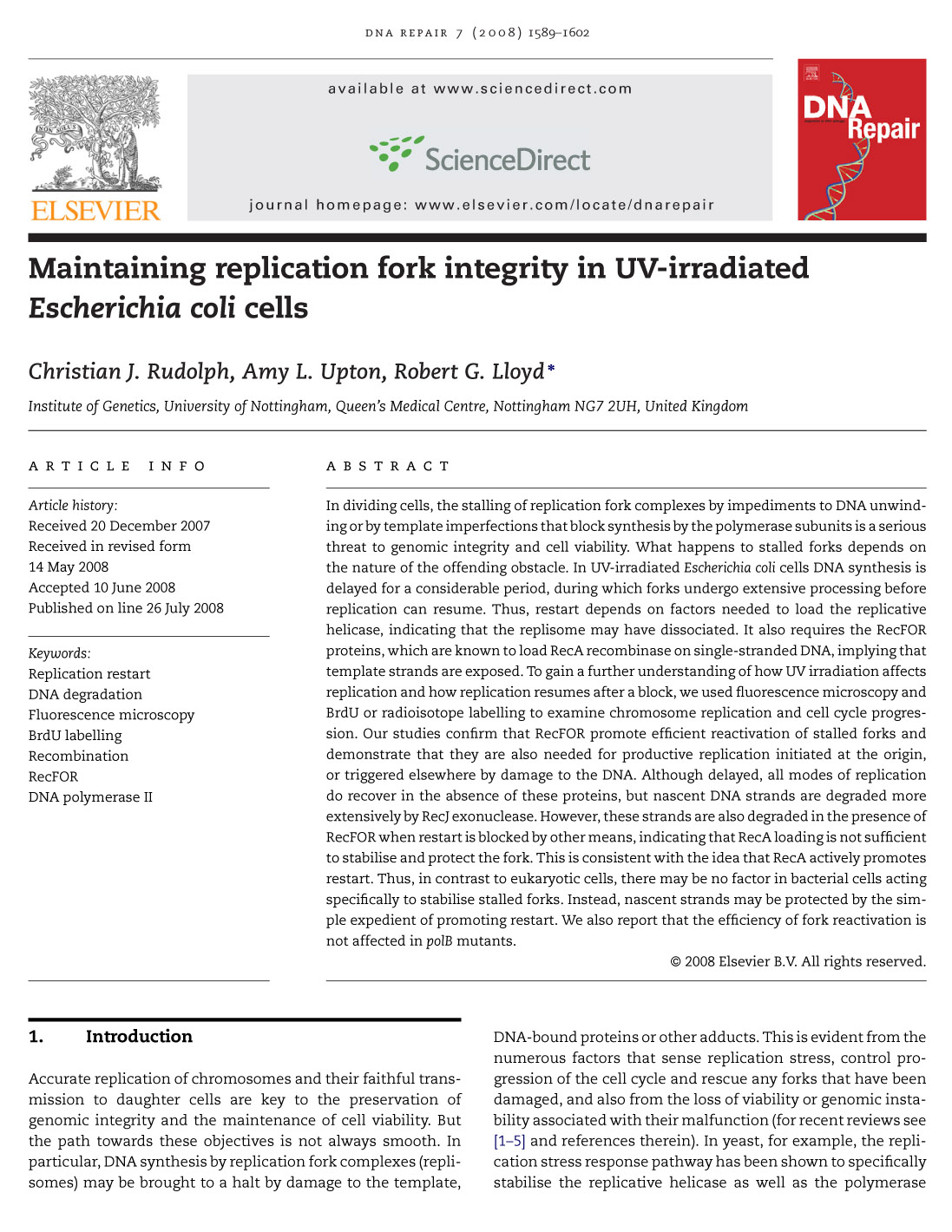The image depicts a scientific journal article from the publication "DNA Repair," Volume 7, spanning pages 1589 to 1602, dated 2008. At the top of the page, prominent elements include the DNA Repair journal logo and the Elsevier logo, which features a tree, alongside the ScienceDirect.com identifier. The article is titled "Maintaining Replication Fork Integrity in UV-Irradiated Escherichia Coli Cells," authored by Christian J. Rudolph, Amy L. Upton, and Robert G. Lloyd from the Institute of Genetics, University of Nottingham, Queen's Medical Center, Nottingham, NG7TU, United Kingdom.

The left margin of the page contains bibliographic information and keywords, detailing the article's history as received on December 20, 2007, revised on May 14, 2008, accepted on June 10, 2008, and published online on July 26, 2008. Keywords for the study include replication restart, DNA degradation, microscopy, BRDU labeling, recombination, RE4 protein, and PALMERS 2 DNA.

A detailed abstract and introduction sections are present but challenging to read in the image. The detailed text and structured content suggest the article focuses on the mechanisms by which E. coli cells maintain the integrity of replication forks following UV irradiation, providing insights into cellular DNA repair processes.